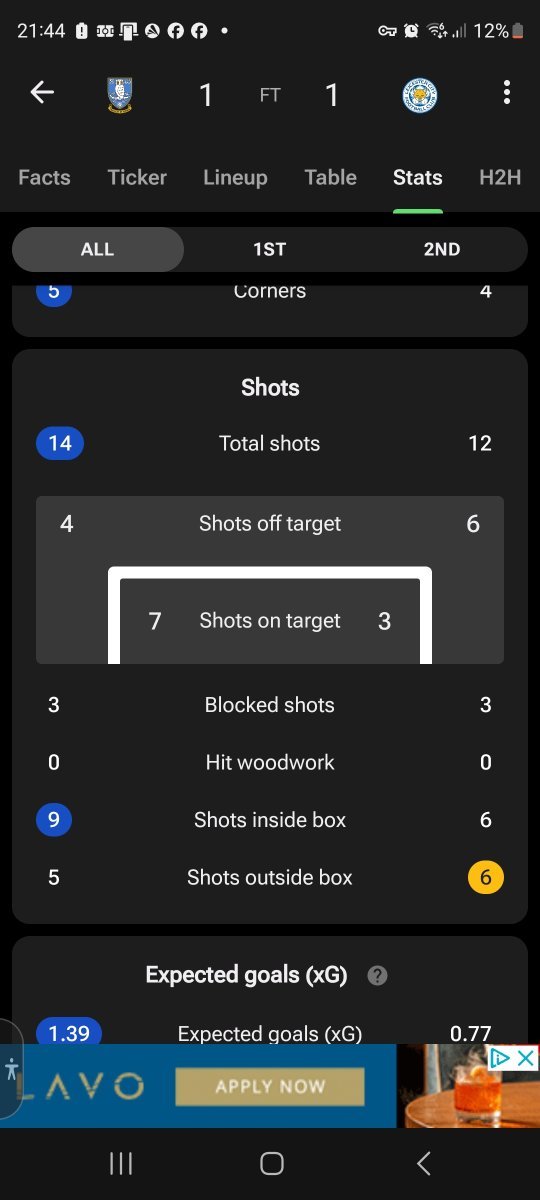The image features a statistical scoreboard against a black background. At the top left, there is a segment labeled "All," though the very top of the image is cut off. In the center at the top, the words "First" and "Second" are displayed, with a blue-highlighted number "5" next to "First." Directly beneath "First" and "Second," the term "Corners" is prominently displayed in the middle of the image, followed by the number "4" on the right.

Center-aligned statistical data flows from the middle outward. The word "Shots" is centrally placed, with the corresponding statistics highlighted in blue. The numbers indicate "14 Total Shots," followed by "12 Shots off Target," "4 Shots on Target," and "3 Blocked Shots." Additionally, "0 Hit Woodwork," "9 Shots Inside Box," and "5 Shots Outside Box" are listed, each followed by their respective values.

Below these figures, the image mentions "Expected Goals" indicated by a symbol "G" and a question mark. Further down, a blue bar with the text "AVO Apply Now" appears prominently. In the lower section, a small coffee table with a red drink is visible.